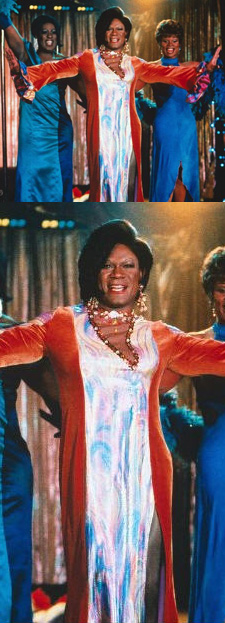The image consists of two screenshots from a movie performance featuring three black men dressed in drag, putting on a vibrant stage show. The larger picture showcases the central performer, who appears as a woman in a striking red dress adorned with white and blue streaks, and wearing large earrings and a bracelet. Her arms are extended outwards, exuding an energetic and charismatic presence. Flanking her on both sides are two backup singers dressed in sleeveless blue silk dresses with matching feathered boas wrapped around their necks. These performers also contribute to the lively atmosphere with their synchronized arm movements. The backdrop features a brown curtain on the left and a golden curtain on the right, enhancing the theatrical setting. The top part of the image is a smaller, zoomed-in version of the same scene, focusing more closely on the lead performer's expressive face and dynamic pose.